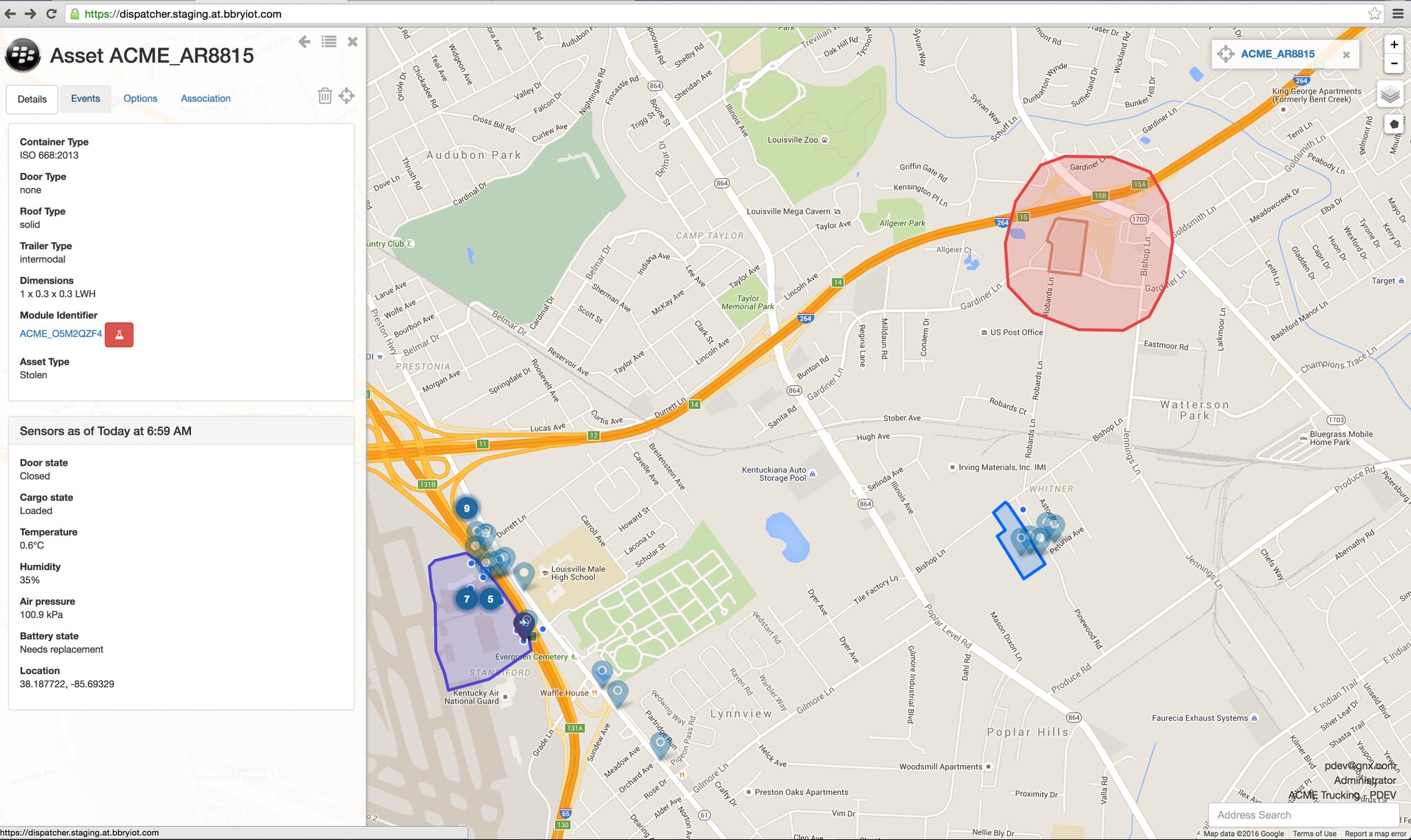The image depicts a detailed map displayed within a web browser at the URL dispatcher.staging.at.bbriot.com. The map highlights various transportation paths, including highways and intersections. Specifically, it marks Exit 131B and Route 264, which branches from the center and progresses to the top-right of the map. A significant area, highlighted with a red circle and a pinkish overlay, indicates a point of interest around Exit 131B, with an additional smaller red outline inside for further emphasis. On the far left side of the map interface, the label "ACME_AR 8815" appears, accompanied by tabs such as Details, Events, Options, and Association, suggesting additional information and control options. At the bottom left, a section titled "Sensors" notes data as of 6:59 a.m., possibly indicating real-time or recent sensor input related to the highlighted area.